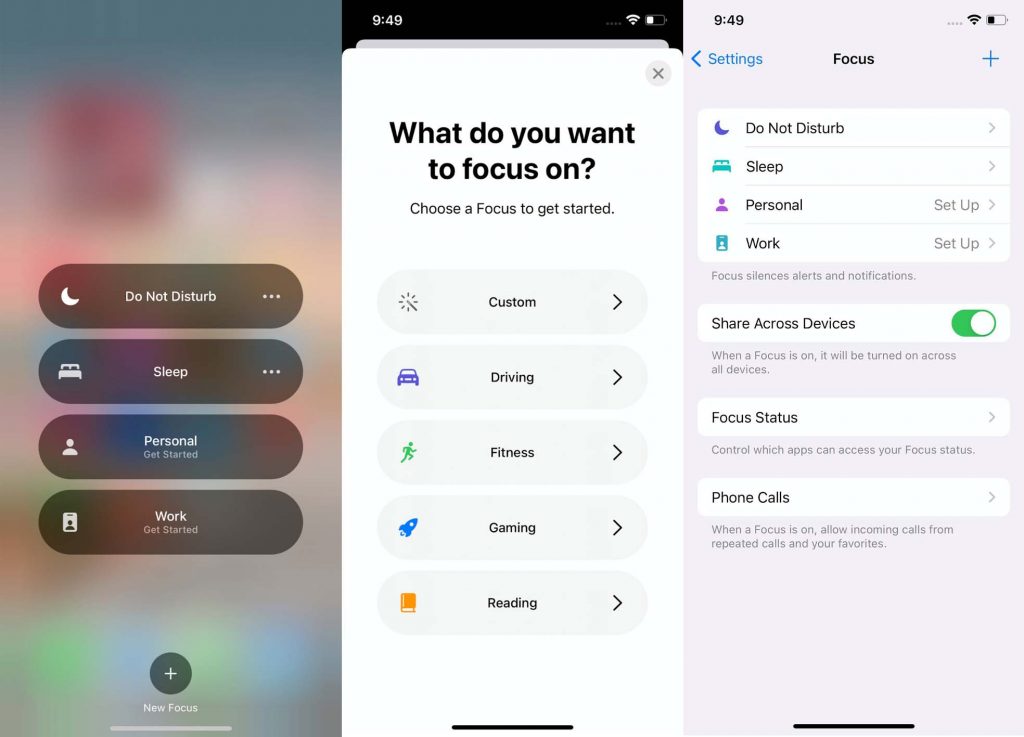The image depicts a smartphone interface for managing focus settings. On the left side, there's an icon representing a bed, indicative of sleep settings, followed by a section labeled "Personal," and "Work." The central part of the image includes a top bar displaying the time "9:49," Wi-Fi status, and a battery icon that is not fully charged.

Below this, text prompts the user with "What do you want to focus on?" followed by customizable options for different focus modes. Categories include:
- Custom
- Driving
- Fitness (highlighted with a blue card)
- Gaming (highlighted with a green card featuring a rocket ship icon)
- Reading (highlighted with an orange book icon)

To the right, there are icons for settings, adding a new focus (+), "Do Not Disturb," Sleep, Personal, and Work modes. 

Further down, the interface lists options related to alerts and notifications:
1. "Share across devices" with a green toggle switch indicating that the setting is on.
2. "Focus Status" detailing control over which apps can access your focus status.
3. "Phone Calls" noting that when a focus mode is on, most incoming calls will be silenced, except for calls from favorite contacts.
  
The overall layout seems to be the settings page specific to configuring various focus modes on a smartphone.